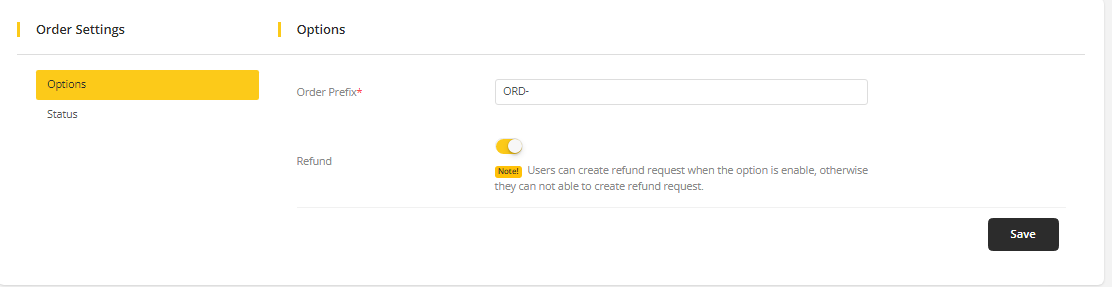This screenshot captures a user interface of a website, featuring a stark white background. The top portion is segmented into two sections: "Order Settings" on the far left, and "Options" to its immediate right. Both section titles are marked by a vertical yellow line to their left. Under "Order Settings," there are sub-options including "Options" and "Status," with "Options" currently selected, highlighted by a yellow-orange rectangular background.

Beneath the "Options" section resides several configurable fields. First, the "Order Prefix" field, which displays a text box containing "ORD-." Below that, there's a "Refund" toggle that is switched on, indicated by a yellow fill. An accompanying note clarifies that when this toggle is enabled, users have the ability to create refund requests; otherwise, they will not have this capability.

In the bottom right corner of the screenshot is a "Save" button with a black background and white text, providing users a clear call to action.